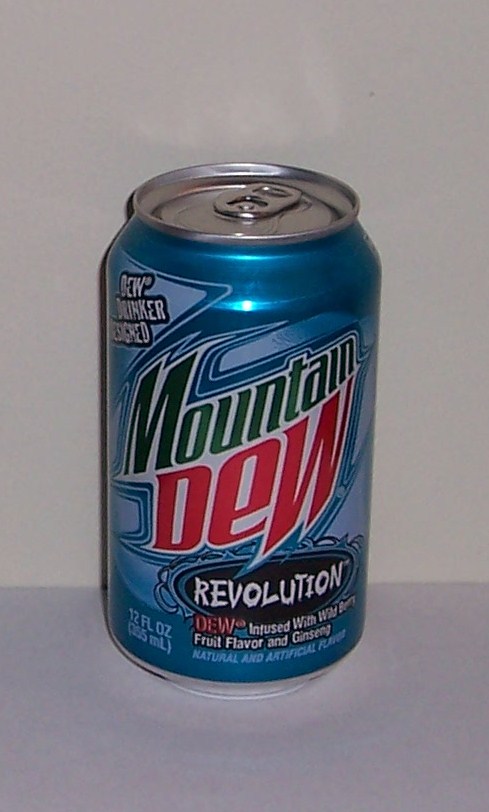This close-up image captures an unopened can of Mountain Dew Revolution set against a cream-colored background. The can's vibrant bluish hue stands out, prominently displaying the Mountain Dew logo in bold green and red letters. Below the logo, the flavor "Revolution" is highlighted in a distinctive font encased within a black oval. Further detailing, the text "Dew infused with wild berry fruit flavor and ginseng" is visible, indicating the blend of natural and artificial flavors. Additionally, the lower left corner of the can specifies the volume as "12 fluid ounces." Shadowed text on the left side of the can is partially obscured.